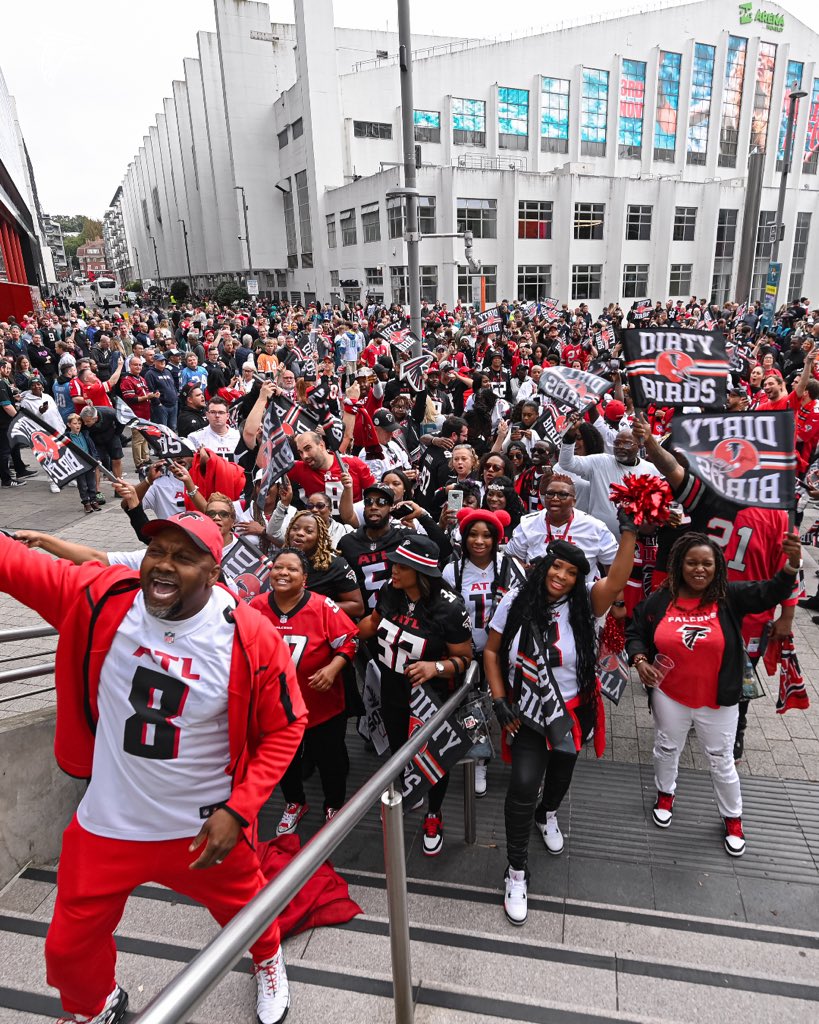This vibrant photo captures a large, excited crowd of Atlanta Falcons fans, either attending a rally, heading to a game, or celebrating a victory. The photographer appears to be standing above on some stairs, capturing the sea of approximately 200 to 300 fans adorned in the team's black, red, and white colors. Many fans are waving flags emblazoned with "Dirty Birds," the affectionate nickname for the team, while others are proudly wearing jerseys featuring various players' numbers and the "ATL" insignia. The fans, wearing a wide array of branded merchandise—including shirts, jerseys, sweatsuits, hats, and even socks—exude energy and excitement. At the forefront of the image, an ecstatic man is seen in a red jersey with the number 8, complemented by red pants, a white shirt, and a Falcons-branded cap. To the right, an African-American woman also stands out, donning an Atlanta Falcons shirt. The backdrop features a building with numerous windows, one prominently displaying a date, "3rd of November," and an image of a woman, adding to the bustling, celebratory atmosphere.